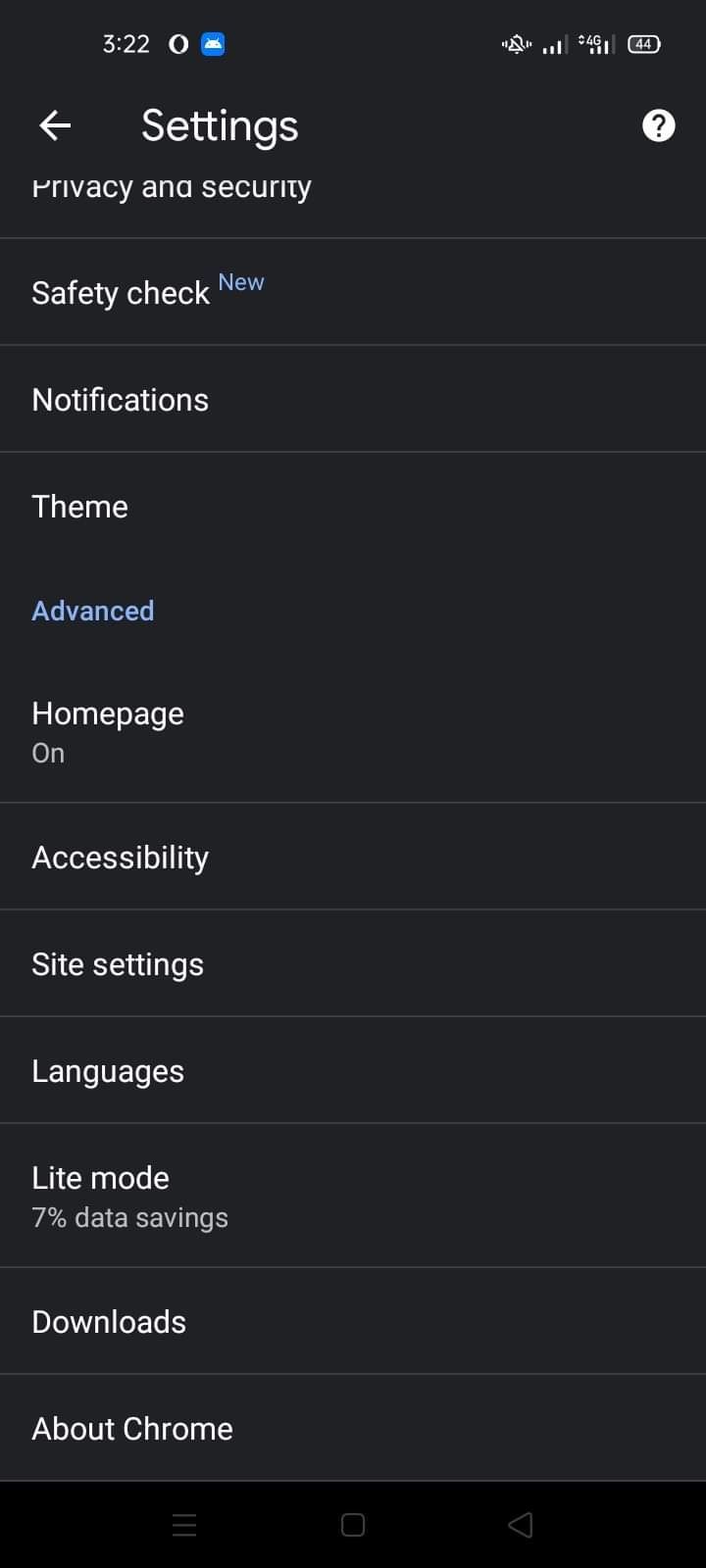The image features a dark grey background with a minimalistic UI design. In the top left corner, the time reads "3:22," accompanied by a signal indicator showing 3 out of 4 bars. Below the time, there's a white arrow pointing left next to the word "sentence." Nearby, a white circle with a grey question mark adds a touch of intrigue.

To the left, "Privacy and Security" is prominently displayed, separated by a light grey horizontal line that extends fully across the width of the image. Beneath this section, "Safety Check" is written, followed by the word "No" in blue text, underlined by another grey line.

Continuing downward, the word "Notification" is written in white, followed by another grey line. Next, the word "Theme" appears in white text, and directly below it, "Advanced" is highlighted in blue.

Further down, the phrase "Home Page" is displayed in white, with the status "On" written underneath it. This is followed by a horizontal line. Below that, "Accessibility" is written, succeeded by another left-to-right line. Farther down, "Sight Setting" appears, followed by a subsequent line.

Towards the bottom of the image, the word "Languages" is displayed, with an additional line beneath it. Finally, the phrase "Light Mode" is shown, with "7% data savings" noted at the bottom.